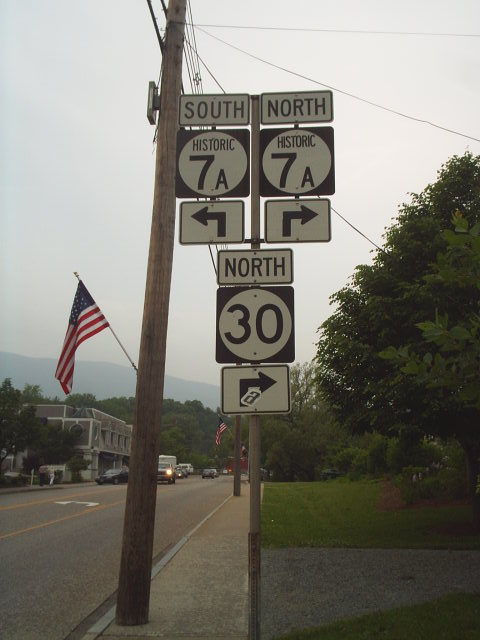In this outdoor color photograph taken during the daytime under a hazy white sky, the main focus is a series of road signs mounted on a single pole. In the center of the image, the pole supports multiple US American roadway signs. At the very top, two rectangular signs display "South" and "North" for historic Route 7A. Just below are two white triangles with arrows, one pointing left and the other right. Further down, there is a white rectangular sign saying "North," beneath which is a black square with a white circle containing the number "30." Below this is another rectangular sign with a right-pointing arrow, partially obscured by a sticker with a lowercase "a."

Adjacent to the left of the pole is a tall brown utility pole with telephone wires and an attached American flag. The scene includes a three-lane road with some vehicles parked along the side. In the midground, there's a two-story building that appears to be a hotel, while to the far right in the background, a fully grown tree with green leaves stands near a patch of grass and a sidewalk. The overall atmosphere suggests a town setting with moderate traffic and a mix of urban and natural elements. The sky is notably overcast, adding to the hazy ambiance of the scene.